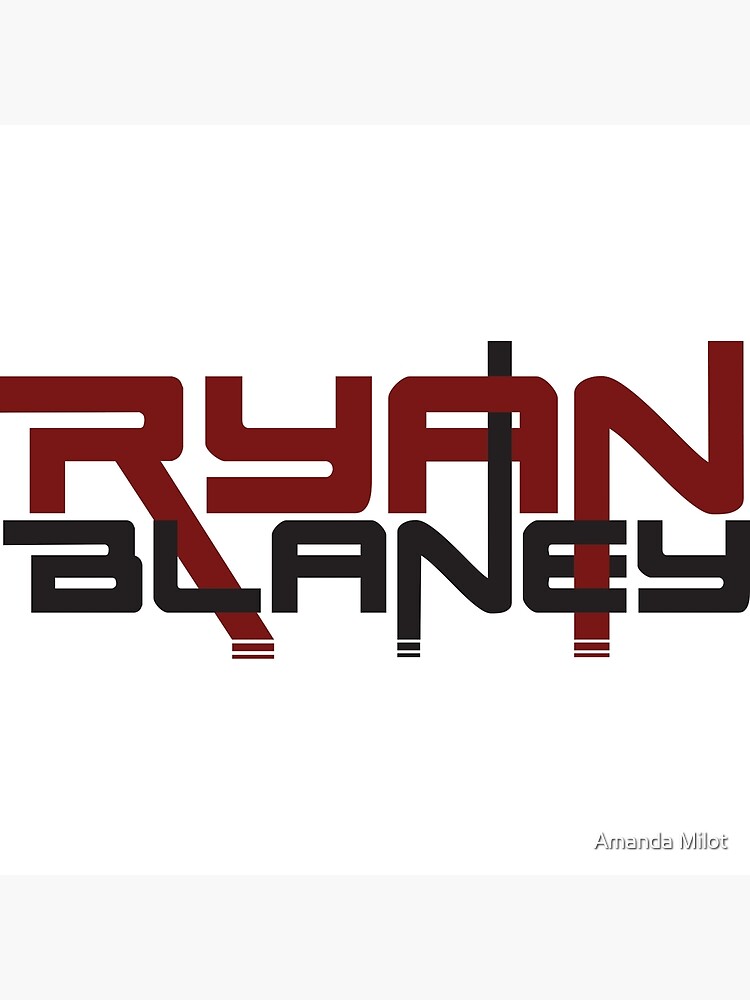The image features a computer-generated sign on a white background displaying the name "Ryan Blaney" in a highly modern, custom-designed, all-caps font. The word "Ryan" is written in red letters, while "Blaney" is in black letters. The typography is unique, with intersecting elements: the bottom right line of the "R" in "Ryan" extends downwards into the word "Blaney," the leftmost vertical line of the "N" in "Ryan" extends downward into the "E" of "Blaney," and the rightmost vertical line of the "N" in "Blaney" extends upwards and intersects through the "A" in "Ryan." Additionally, in the bottom right corner of the image is a watermark that reads "Amanda Milot."